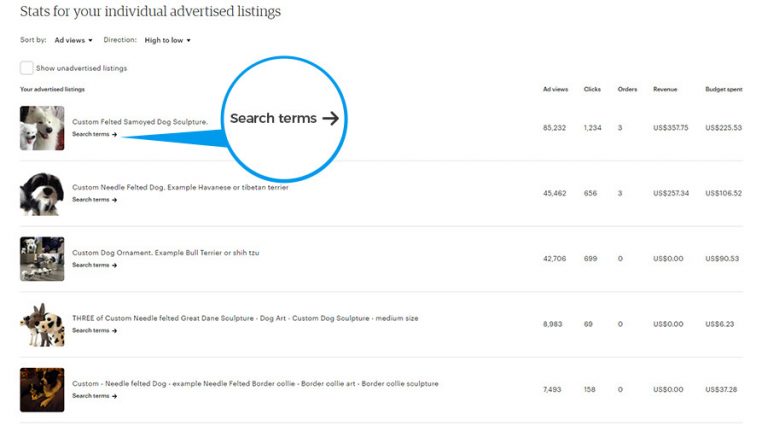This image showcases a detailed analytics screen for individual advertised listings. On the left side, there is a list of five different product names, each accompanied by a thumbnail image of various types of dogs. Adjacent to each product name and image, there are five statistical categories displayed: ad views, clicks, orders, revenue, and budget spent. These statistics are presented in gray text, aligning with their corresponding listings. The right side of the screen features a notable blue circle around the section labeled "search terms," with an arrow pointing to the detail categories on the right. The entire layout is set against a clean, white background, enhancing readability and organization.